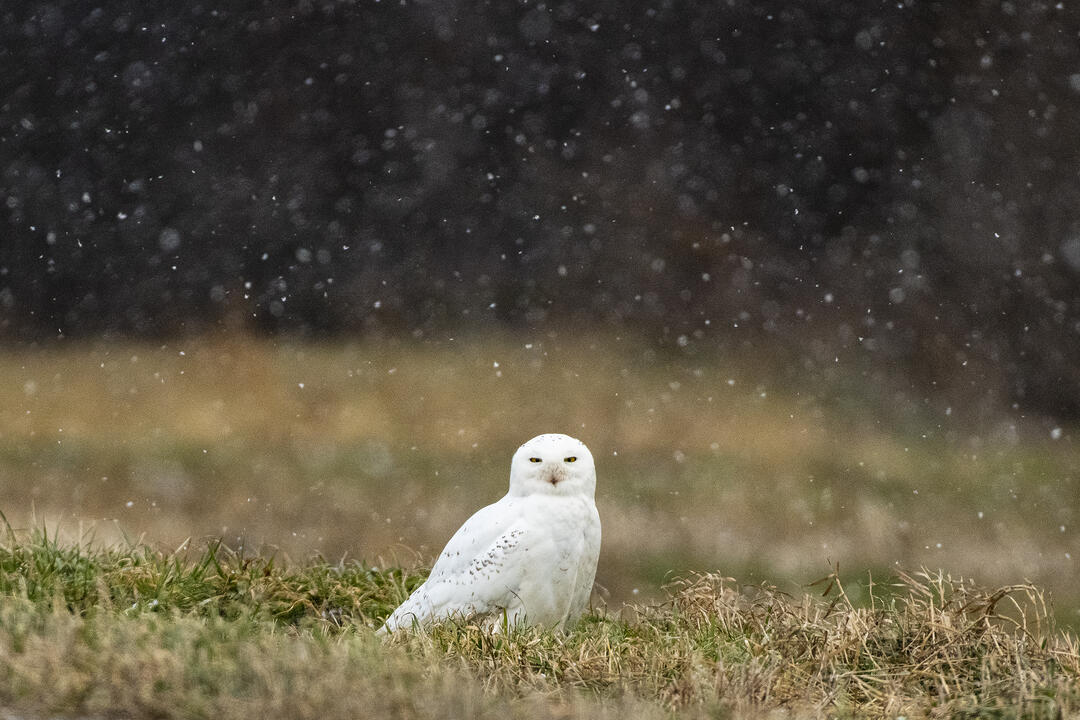In this captivating photograph, a striking white owl takes center stage as it stands in an open grass field under a gentle snowfall. The owl is the clear focus of the image, with its pure white feathers contrasted by a few distinct black spots on its wings. Light tan and black eyes accentuate its gaze, which is fixed directly at the camera, and a small brownish beak completes its sharp features.

The grass surrounding the owl is a mix of green and yellowish-brown, indicative of a wintry landscape where some vegetation is beginning to die off. Despite the falling snowflakes, no significant accumulation is evident on the ground, allowing the patchy grass to remain visible. The background of the image features more of this grassy field, which fades into a dark, blurred backdrop that likely contains trees, although they are difficult to distinguish due to the pronounced bokeh effect. The overall scene evokes a serene yet mysterious atmosphere, with the wintry elements enhancing the owl’s ethereal presence.